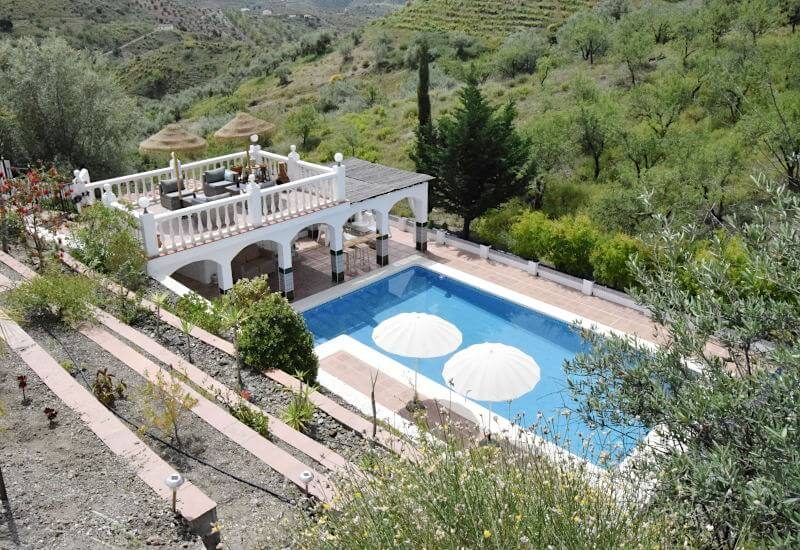The aerial view captures an impressive outdoor entertainment area of an elegant villa nestled in a hilly landscape. The centerpiece is a large, horizontally rectangular, built-in swimming pool with bright blue water sparkling under the sunlight. Two sizable, round white floats drift on the water’s surface. The pool is bordered by a white stone or cement edging and surrounded by a tiled brick patio walkway. At the lower right of the pool, the land slopes steeply, meticulously landscaped to blend with the natural surroundings, while treetops frame the scene.

Elevated prominently on the upper left side of the image is an elegant deck featuring a white railing, lounge furniture, umbrellas, and two gas-powered barbecues, creating a perfect spot for relaxation and outdoor dining. This deck, supported by an arched portico with high arches, extends from a stone incline. Underneath the deck, the tiled brick area continues, offering a shaded space for various activities.

The background reveals rolling hills adorned with green grass, vegetative shrubs, and tall conifer trees. The landscape also features grapevines and trails, further emphasizing the villa's luxurious setting amidst a serene valley. The villa’s sophisticated architecture and well-manicured surroundings seamlessly integrate with the natural beauty of the hills.